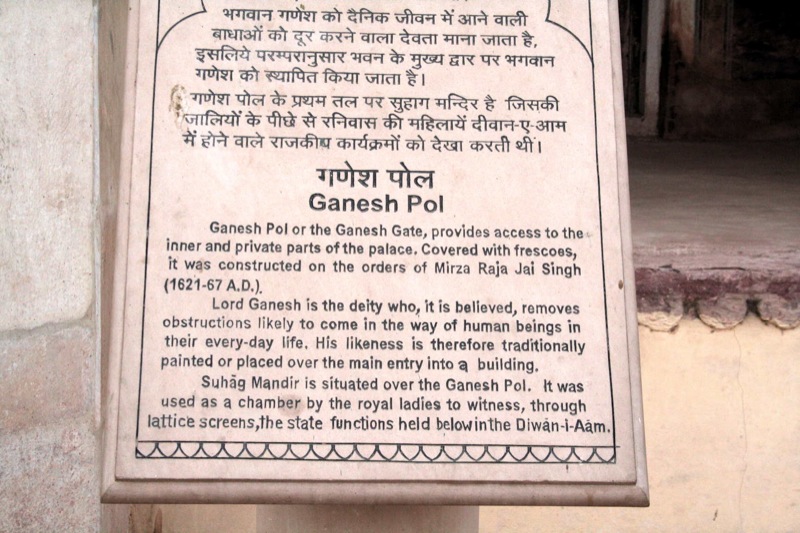The image depicts a rectangular, aged stone plaque with inscriptions in both a foreign language and English. The top part of the plaque features text in an unfamiliar script, while the rest is written in black English letters on a discolored white stone. The plaque reads "Ganesh Pol," which translates to "Ganesh Gate." The description explains that the gate allows access to the palace's inner and private sections and is adorned with frescoes. Constructed on the orders of Mirza Raja Jai Singh between 1621 and 1667 AD, the plaque highlights the significance of Lord Ganesh, regarded as the remover of obstacles in daily life, whose image is traditionally placed above main entrances. Additionally, the plaque mentions Suhag Mandir, a chamber above the Ganesh Gate used by royal ladies to observe state functions through lattice screens within the Diwan-i-Am. The plaque itself is mounted on a small support in front of a stone building wall, hinting at a historical and cultural setting.